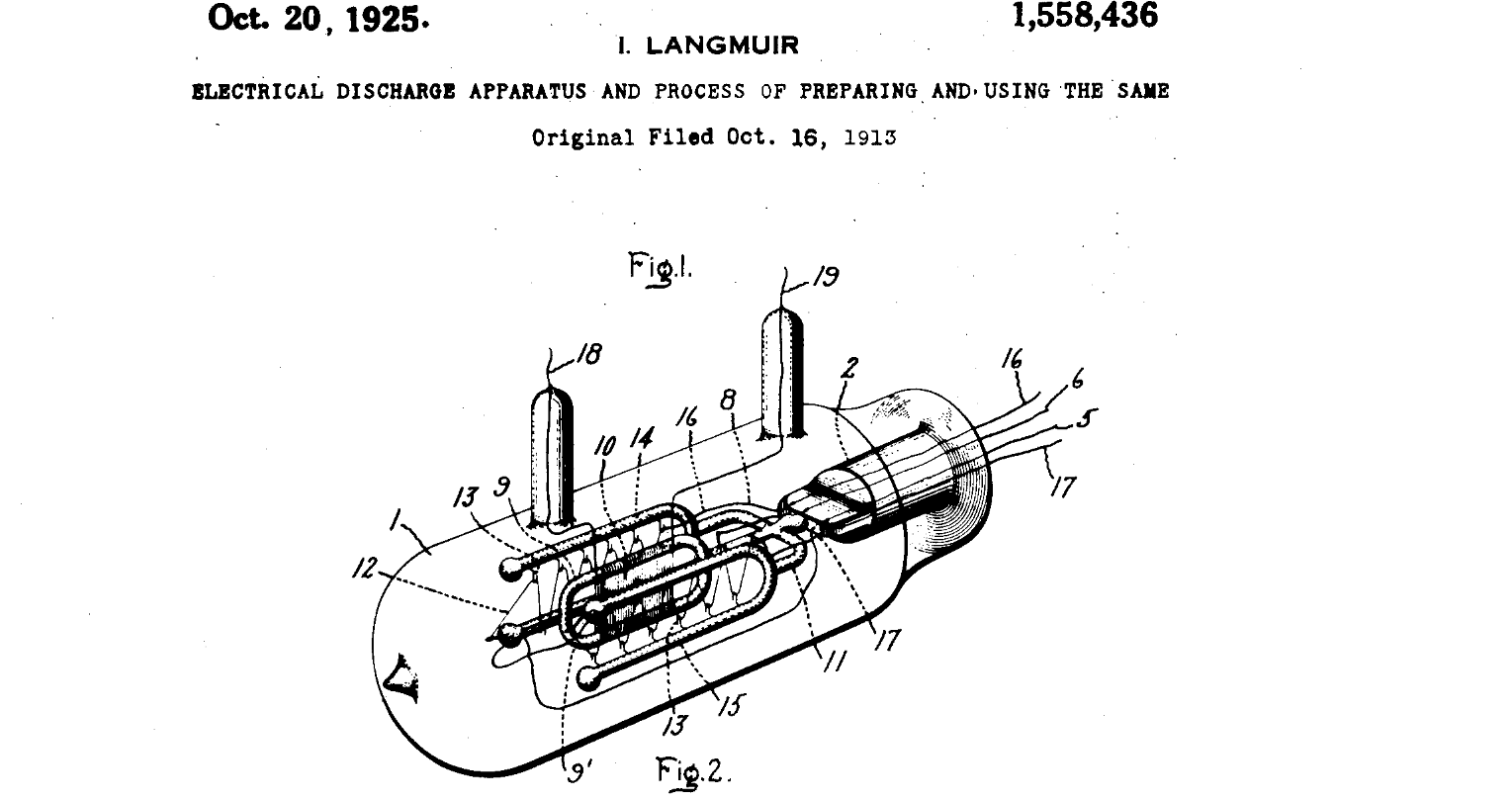The image presented is a detailed, black-and-white schematic drawing that bears a strong resemblance to an old-style light bulb or a similar electrical discharge apparatus. The background is the plain white of a screen, emphasizing the clear and bright setting of the image. Prominently displayed in black text at the top of the image is the date October 20, 1925, in the upper left corner, the number 1,558,436 in the upper right corner, and the name I. Langmuir centered at the top. Below this, the text reads: "Electrical Discharge Apparatus and Process of Preparing and Using the Same," followed by "Original filed October 16, 1913."

The central illustration depicts a tapered tube featuring intricate internal twists and turns. The tube's configuration suggests a classic light bulb structure, with projections or pegs protruding from both the front and back ends. The schematic style of the illustration includes numerous labeled parts, with numbers ranging up to 19, although the specific meanings of these numbers are not provided. The figure is divided into two sections labeled "Figure 1" at the top and "Figure 2" below it. Overall, the precision and annotations lend an air of technical documentation to the image, reflecting its historical and scientific significance.